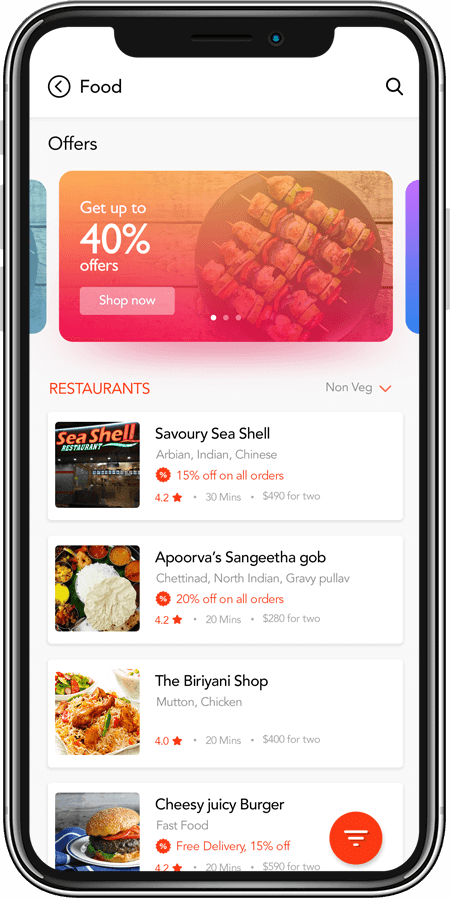Screenshot of a Mobile App:

The screenshot showcases the interface of a mobile application. On the left side of the phone, the volume button is visible, while the on/off button is located on the right side.

The top section of the screen features the heading "Food", followed by a subheading that says "Offers". An orange box prominently displays the text "Get up to 40% offers". Beneath this message is a pink "Shop Now" button. Inside the orange box, there's an image of kebabs arranged on a plate.

Below this promotional section, a heading in uppercase orange text reads "RESTAURANTS". Four restaurant listings are presented, each accompanied by specific details:

1. **Savory Shell**: Offers Arabian, Indian, and Chinese cuisine with a 50% discount. It has a rating of 4.2 stars and an estimated delivery time of 30 minutes. The average cost for two people is approximately ₹490.

2. **Purva's Sanjita Gob**: Provides a 20% discount on all orders. It is rated 4.2 stars, with an estimated delivery time of 20 minutes and an average cost of ₹280 for two people.

3. **The Biryani Shop**: This restaurant has a 4-star rating, an estimated delivery time of 20 minutes, and an average cost of ₹400 for two people.

4. **Cheesy Juicy Burger**: Offers free delivery and a 50% discount. It boasts a rating of 4.2 stars, requires around 20 minutes for delivery, and costs approximately ₹590 for two people.